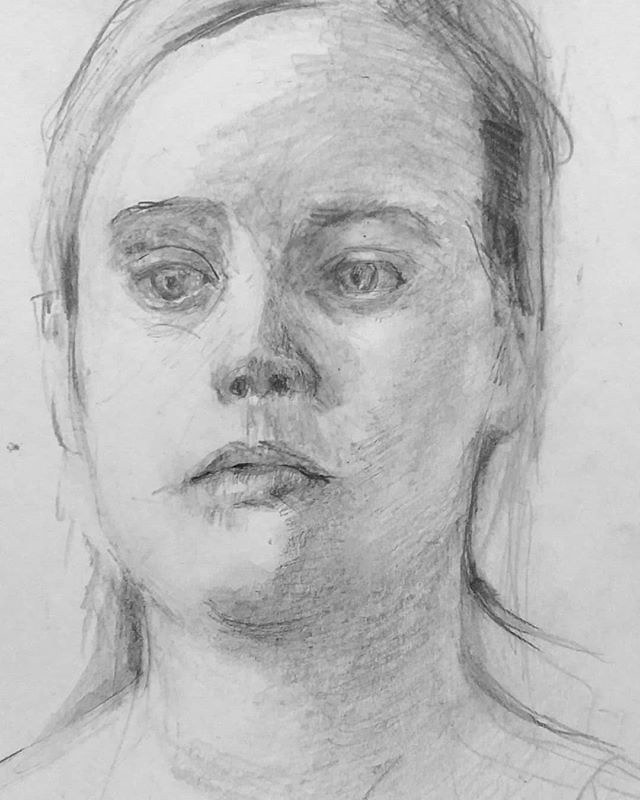A detailed, shaded pencil sketch on textured craft paper depicts a young blonde woman looking solemnly to the left. Her thin, long hair cascades down the left side of her face, while the right side appears pulled back, possibly by a barrette. The drawing captures her head, neck, and partially her shoulders, showing her serious, somewhat sad expression. The artist skillfully employs various shading techniques to bring depth to the monochrome depiction, highlighting the woman's delicate features and vacant gaze, suggesting thoughtful contemplation. The high-quality execution of the sketch indicates the artist's considerable talent and practiced hand.